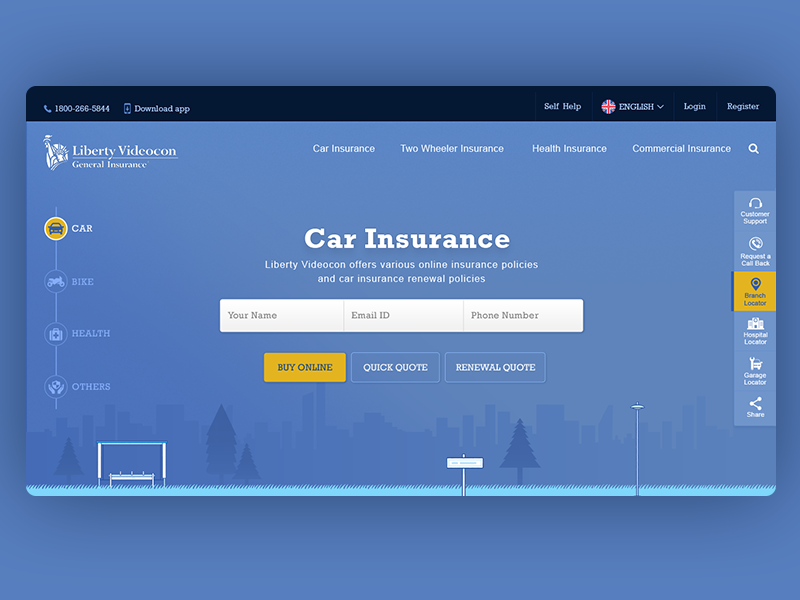This screenshot captures the homepage of the Liberty Video Con Core Insurance website. At the very top, there is a sleek black bar featuring a contact phone number, a prompt to download their app, and four action buttons aligned to the right. Directly below, the website exudes a lighter blue hue. In the upper left corner, the logo prominently displays the Statue of Liberty, with "Liberty Video Con" underlined, and "General Insurance" written beneath it.

Adjacent to the logo, on the right, is the top navigation bar for easier site exploration. Centrally, the site title "Core Insurance" is boldly presented in large white text, with a smaller white tagline beneath it that reads, "Liberty Video Con offers various online insurance policies and car insurance renewal policies."

The main section of the page features three distinct data-entry fields, each outlined in white. These fields are labeled for users to input their name, email ID, and phone number, thereby facilitating user interaction and engagement with Liberty Video Con's online services.